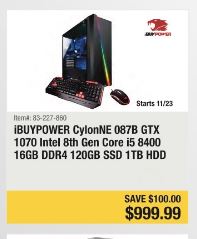This image appears to be an online advertisement for a gaming computer, resembling a slightly rectangular, almost square screenshot. The ad is bordered by a gray frame. The upper half of the image features a white rectangle displaying a photograph of a black desktop computer. The computer is illuminated with blue lighting visible inside its casing. Accompanying the computer, there is a keyboard positioned in front of it and a black mouse to the right side. Below this, the item number "832-27880" is inscribed. The product is labeled as "iPower Cyclone NE 0870GTX 1070," equipped with "Intel eighth generation Core i5 8400" processor. In the bottom right corner of the ad, the price is listed as "$999.99." Directly above this price, a yellow rectangle highlights a promotional message, stating "Save $100."